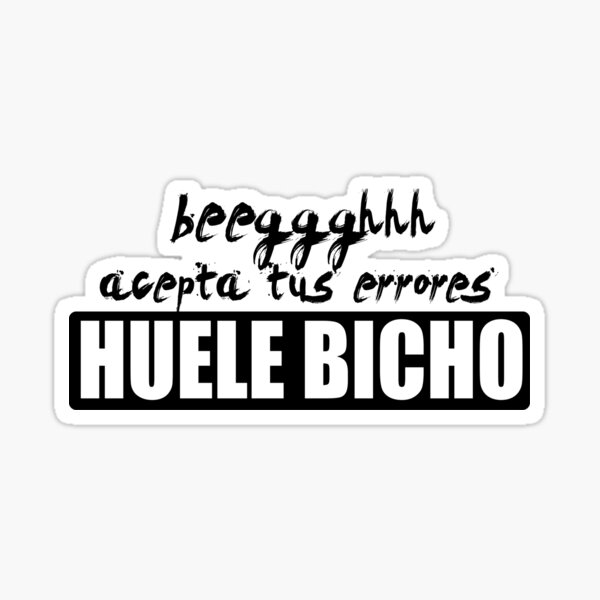The image is rectangular, slightly taller than wider, with a predominantly light gray background. Centered within is a sticker or sign-like object featuring black, handwritten-style text that reads "BEEGGGHHH" at the top. Below this, in a similar font, is the phrase "ACCEPTA TUS ERRORES." The bottom section of the sign features bold white, uppercase text stating "HUELE BICHO" set against a black rectangular background. The entire composition is bordered by a cloud-like outline that adds a distinct separation from the background. The image is clear, well-lit, and easy to read.